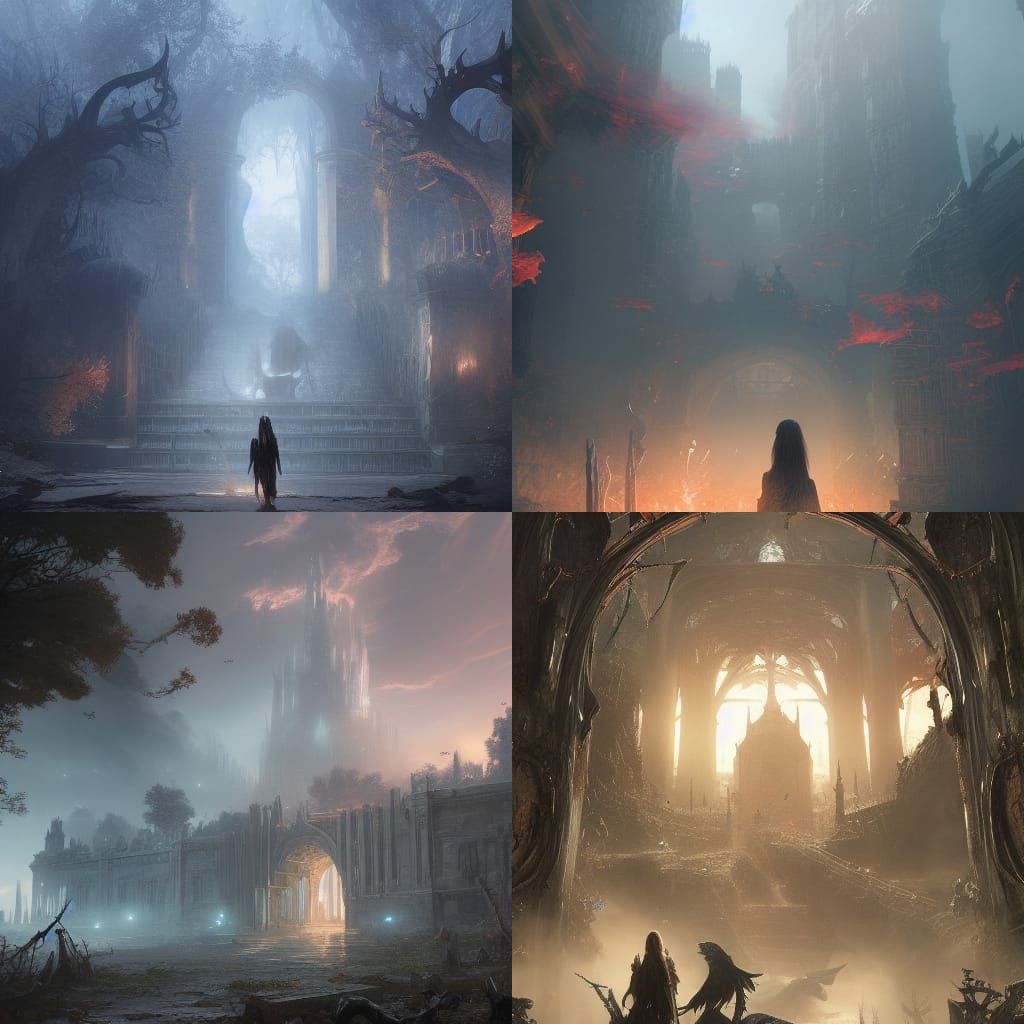This image set comprises four eerie, fog-shrouded scenes reminiscent of a dark, atmospheric video game. The top-left image reveals a long staircase flanked by gnarled trees and bathed in a muted, almost sinister light, with a solitary figure poised to ascend. Adjacent, the top-right image zooms in on this figure moving toward a circular, orange-lit area, intensifying the scene's otherworldly, red-tinged gloom. In the lower-left, we observe a foreboding low building with a large archway, set against a backdrop of towering, spiral structures enveloped in the same eerie mist. Completing the sequence, the bottom-right depicts an arched branch structure framing a building that looms ominously with glowing yellow light amidst surrounding destruction, enhancing the overall sense of desolation and mystery.